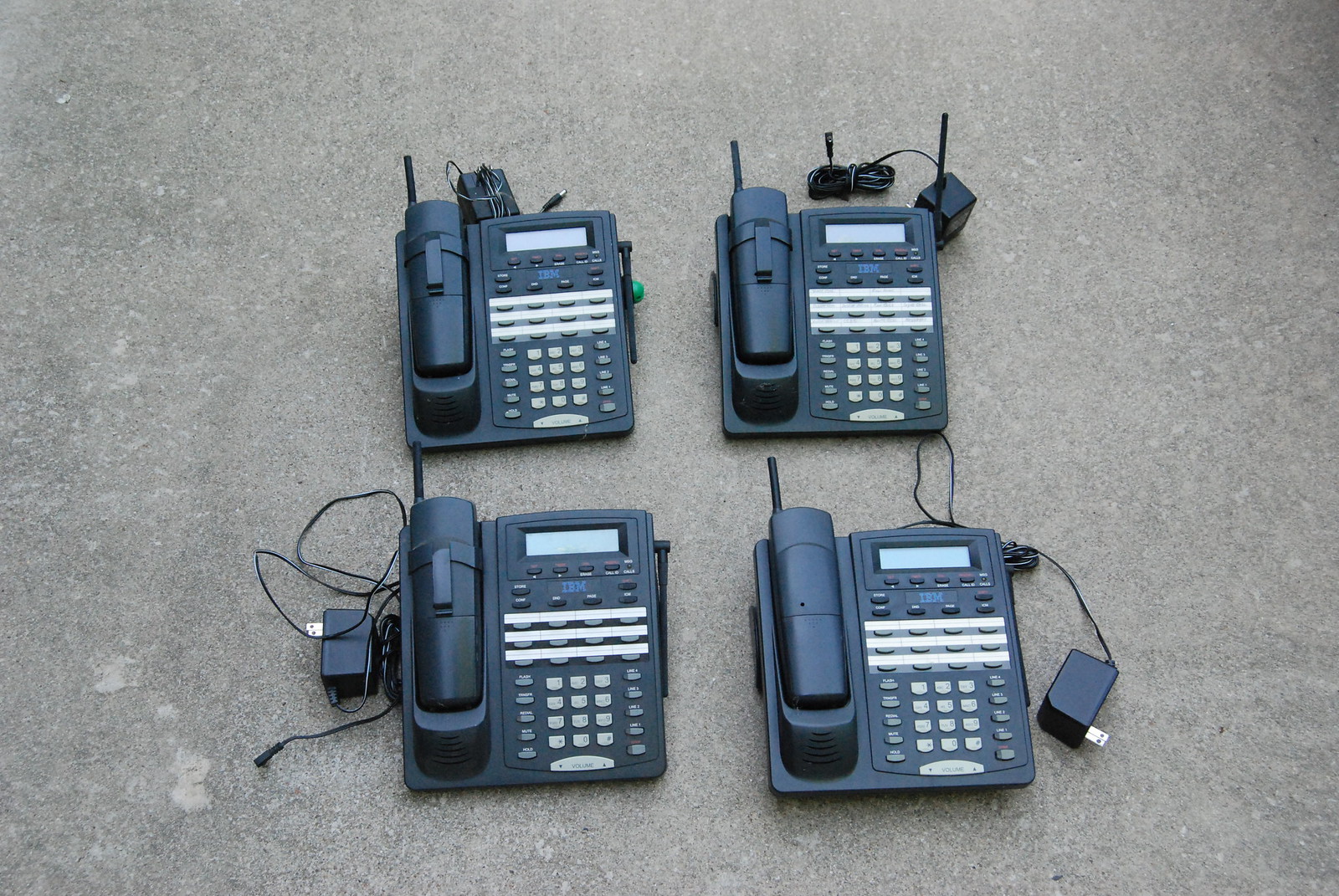This photograph showcases four identical black office-style telephones arranged in a neat grid pattern with two rows of two phones each, all set against a gray, pebbly concrete background. The telephones, reminiscent of older models from the 1980s or 90s, are characterized by their square bases and cordless handsets which feature small antennas—the first, third, and fourth phones having their antennas down, while the second phone’s antenna is up. Each phone includes a digital readout screen for caller identification, numerous gray buttons with varying shades, and three distinctive white lines across the front of the base. Beside each phone, there is a black cord, presumably for connection, with three out of the four handsets sporting a belt clip or similar plastic attachment on the back—excluding the phone in the bottom right corner. These larger, big-button telephones evoke a bygone era, highlighting their practical design tailored for office use.